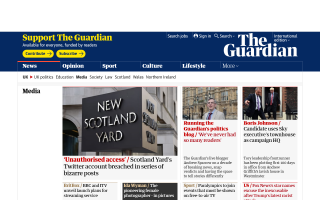The image depicts a webpage from The Guardian, an online news platform. The top of the page features a prominent blue banner that says "Support The Guardian." On the far right of this banner, the publication's name, "The Guardian," is displayed in white letters.

Below the banner, the navigation bar offers several tabs for users to explore: "News," "Opinion," "Sport," "Culture," "Lifestyle," and a "More" option for additional categories. The "News" tab is highlighted with a red underline, indicating it is the currently selected section.

The main body of the page showcases several news articles, although the text is somewhat difficult to read. One of the articles includes an image of New Scotland Yard with a headline reading, "Unauthorized Access: Scotland Yard's Twitter Account Breached in a Series of Bizarre Posts." Another article features an image of a man in front of what appears to be an ancient building, though the details are unclear due to the readability issues. Additionally, an image of a man resembling Donald Trump is present, but again, the text is not legible.

The overall design of the page is predominantly white, providing a clean and uncluttered background that highlights the various news stories and the blue banner at the top.